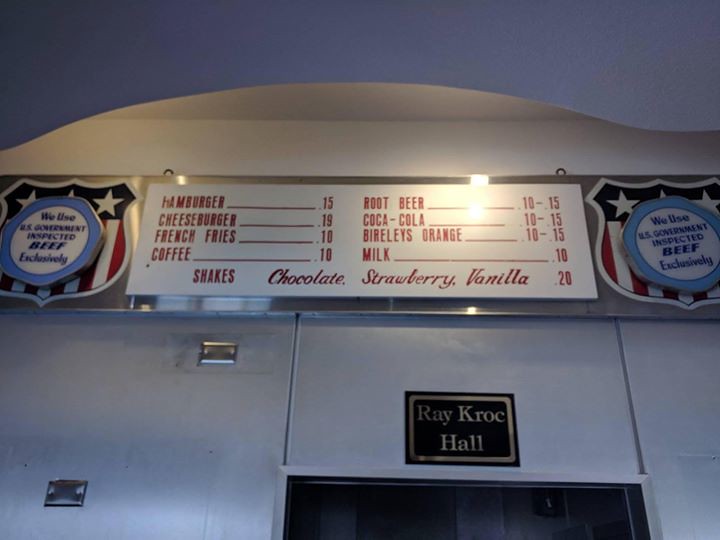The image captures the entryway to "Ray Kroc Hall," a noteworthy section of what appears to be a sports facility. The photograph is taken from a low angle, directed upwards, encapsulating both the entrance and the serene twilight sky. The building's façade is predominately white, providing a stark contrast to the deep blue evening sky above.

Situated centrally at the bottom of the image, slightly off-center to the right, is the top of a black doorway. Hanging above this doorway is a black plaque with a copper border, engraved with the words "Ray Kroc Hall."

Above the plaque, there's a prominent horizontal sign with a metallic silver background. This sign is flanked on both sides by shield-shaped USA flag motifs, each featuring a blue circle in the middle with inscriptions indicating that the facility uses "U.S. Government Inspected Beef Exclusively."

The main section of the sign displays a menu, divided into two columns. The left column lists:

- HAMBURGER: 0.15
- CHEESEBURGER: 0.19
- FRENCH FRIES: 0.10
- COFFEE: 0.10

The right column features:

- ROOT BEER: 0.10
- COCA-COLA: 0.15
- BIRELLI'S ORANGE: 0.15
- MILK: 0.10

Below these, in bold red capital letters, the menu offers:

- SHAKES: Chocolate, Strawberry, Vanilla - 0.20

This detailed entrance and menu signage reflect a nostalgic glimpse into the historical ambiance of "Ray Kroc Hall," likely a cherished landmark within the facility.